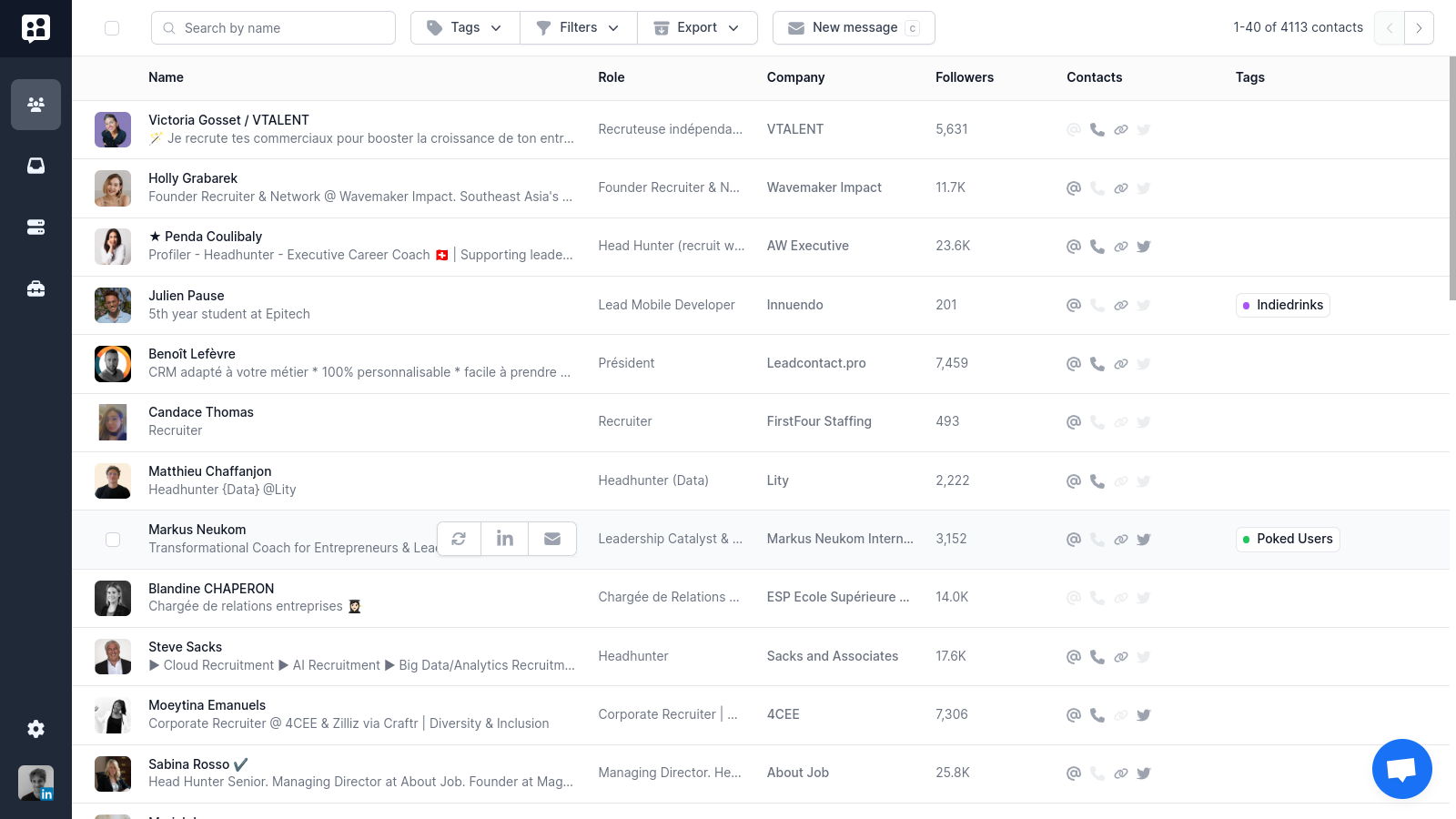This image depicts a webpage with a complex layout containing multiple sections, images, and text. 

On the top left of the page, there is a vertical menu featuring several buttons, each with distinct icons. From top to bottom, these buttons include:
1. A button showing two people.
2. A button showing three people.
3. A button shaped like a square.
4. A “More” button.
5. A button shaped like a suitcase.
6. A settings icon at the bottom.

Beneath these buttons, there is a black-and-white image of a person. The image includes a LinkedIn icon on the bottom right corner of the photo.

In the top middle of the page, there is a search bar with the placeholder text "search by name." 

To the right of the search bar, a horizontal menu displays several tabs, arranged from left to right as follows:
1. Tags
2. Filters
3. Export
4. New Message

Below this menu, the page is divided into multiple sections listing different categories. These categories, displayed from left to right, include:
1. Name
2. Role
3. Company
4. Followers
5. Contacts
6. Tags